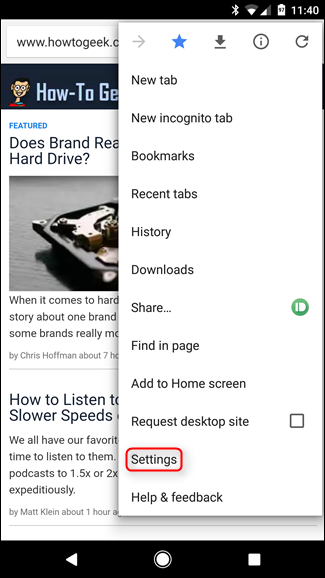**Detailed Caption:**

The image appears to be a screenshot from either a tablet or a smartphone, as indicated by the icons visible at the top of the screen. At the top left, there is a battery icon displaying 97% charge. Next to it, the time is shown as 11:40. Wi-Fi signal, mobile data signal, and Bluetooth icons are also visible on the status bar, signifying the device's connectivity status.

A dropdown settings pane is open on the screen, displaying several options. At the top of this pane, there are icons including a star for bookmarks, a download button, a circular information icon (i), and a back button (arrow pointing left). Below these icons, various menu options are listed: "New tab," "New incognito tab," "Bookmarks," "Recent tabs," "History," "Downloads," "Share" (accompanied by a green and white button), "Find in page," "Add to home screen," "Request desktop site" with a checkbox next to it, "Settings" (highlighted in red, suggesting the user should select this option), and finally, "Help and feedback."

In the background, partially obscured by the settings pane, is a webpage from howtogeek.com. The visible part of the webpage features an image of a hard drive and a headline for a featured article which begins with "Does brand..." although the rest of the headline is not visible. The article's author is Chris Hoffman, and the publication time is noted as approximately seven hours ago.

Overall, the image seems to aim at instructing viewers on how to access the settings menu on an Android device while navigating through a web browser.